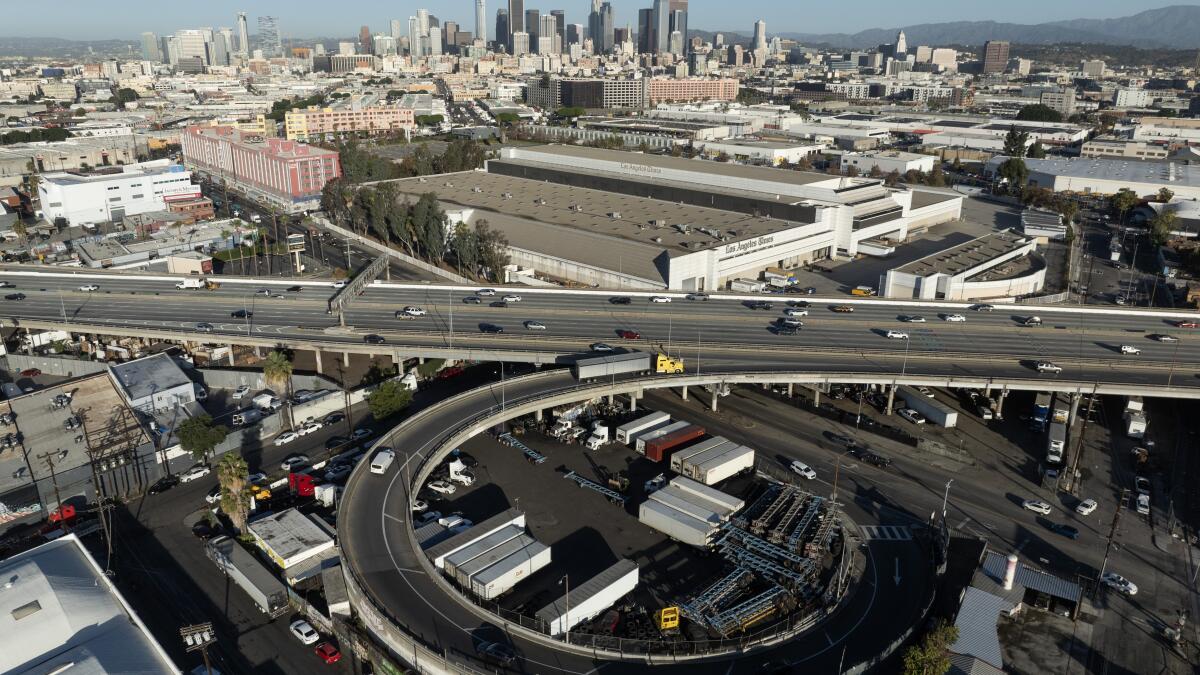An aerial view of a bustling highway showcases a gray roadway packed with numerous vehicles. The cars, a mix of yellow and various other colors, create a vibrant pattern as they move along the route. The road curves inward, forming a noticeable circular shape that adds a dynamic element to the composition. In the top part of the image, several towering skyscrapers dominate the skyline, providing a striking contrast to the busy highway below. The intricate interplay of urban architecture and constant motion captures the essence of city life.